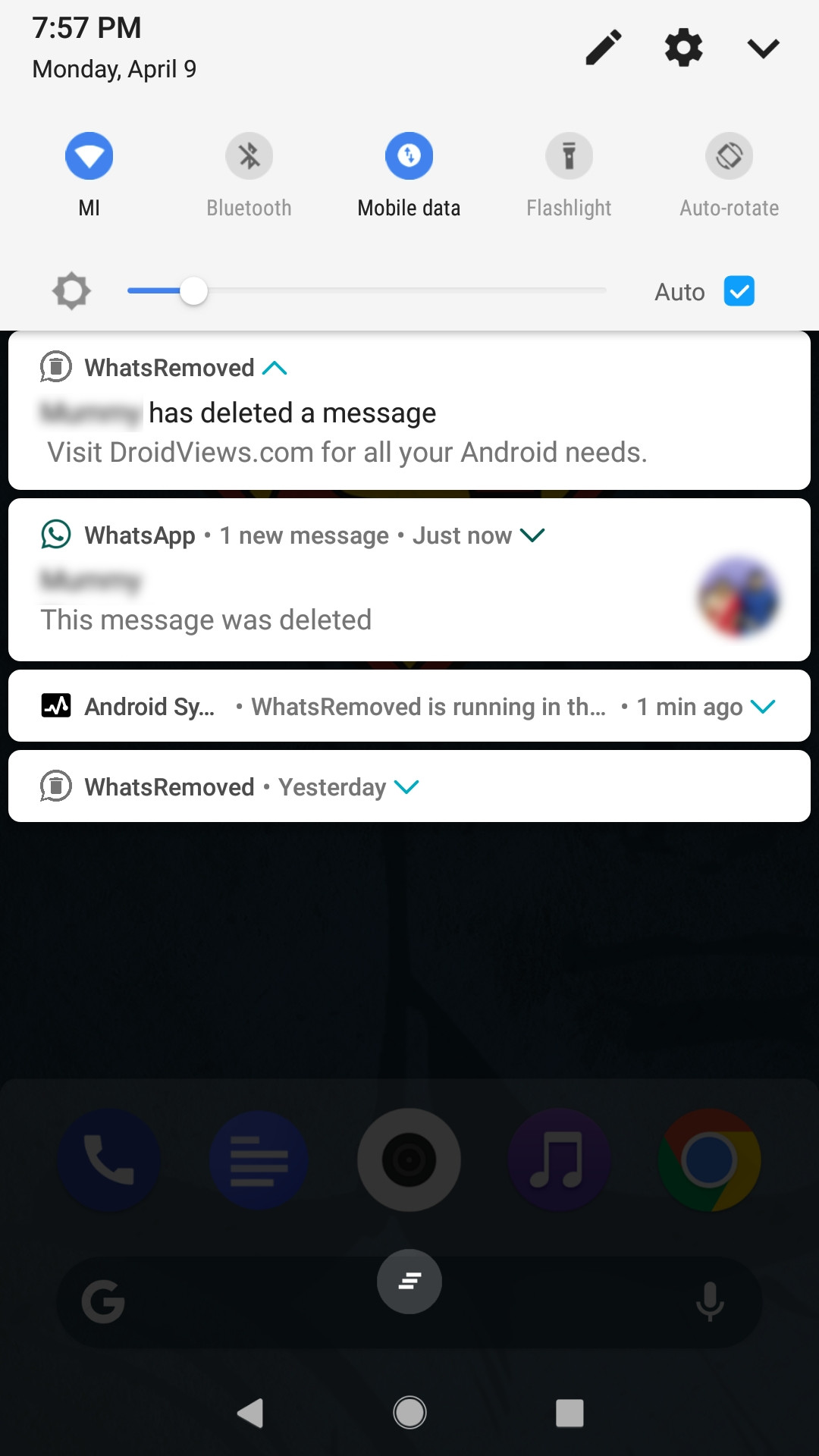The image is a screenshot from a cell phone displaying various notifications and quick settings on the screen, taken while the user had a message recovery app called "WhatsRemoved" installed. 

At the very top, the status bar shows typical icons: a circular 'MI' symbol resembling a Wi-Fi icon, a Bluetooth symbol, a mobile data indicator, a flashlight icon, and an auto-rotate icon. Below this, there's a brightness adjustment bar with a sun icon in gray. The bar features an auto-brightness setting with a blue section on one end, transitioning to a faint gray, and a white checkmark in a blue box indicating activation of the auto feature.

Beneath these icons and settings, a notification from the "WhatsRemoved" app states that a message has been deleted, reading: "What's Removed has deleted a message. Visit droidviews.com for all your Android needs." Additionally, a blurred-out WhatsApp notification indicates a new message with the note "This message was deleted."

Further down, there is another notification partially visible that starts with "Android SY..." and a "WhatsRemoved" notification from the previous day. The bottom portion of the screenshot has a muted black-gray color owing to the blurred-out messages and the overlaying notifications.